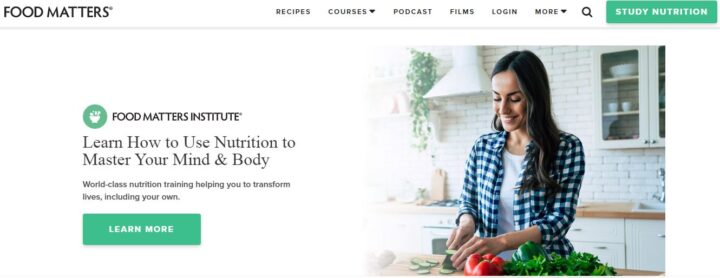This image is a detailed screenshot of a website, likely captured from a laptop in landscape mode. The website features a predominantly white background. At the very top, spanning from the upper left to the upper right, is a white navigation bar.

Starting from the upper left corner, there is a logo displayed in dark black capital letters reading "FOOD MATTERS". Following the logo, the navigation menu includes the categories: Recipes, Courses (with a black downward-facing triangle next to it), Podcasts, Films, Login, and More (also with a black downward-facing triangle). Adjacent to these headers is a search icon and a prominent green button labeled "Study Nutrition".

Below this navigation bar, the left side features a text header in bold that reads "Food Matters Institute." Beneath it, a sub-heading states: "Learn how to use nutrition to master your mind and body. World-class nutrition training helping you to transform lives including your own." Directly underneath this text is another green button that says "Learn More".

On the right side of the page is a large, professional photograph of a young woman in a kitchen. The background of the kitchen includes a cabinet with glass doors in the upper right corner. The woman is dressed in a white shirt with a blue and white plaid cover-up. She is shown slicing cucumbers on a tabletop, with both her right and left hands visible in the action.